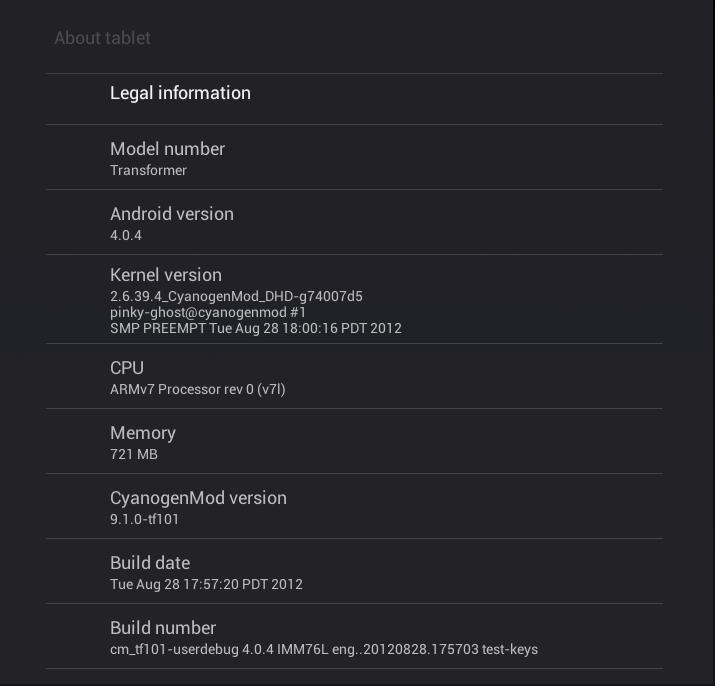This screenshot captures a detailed view of the "About Tablet" section in the settings of a device running a customized version of Android. At the top left, the heading "About Tablet" is displayed in gray text. Below it, the section titled "Legal Information" appears in white text.

Moving further down, the "Model Number" is listed as "Transformer" in gray text. The "Android version" is specified as 4.0.4. Continuing down, "Kernel version" is shown in gray text with detailed information: "2.6.39.4_CYANOGENMOD_DHD-G74007D5." This is followed by a note indicating "Pinky/Ghost@Cyanogenmod #1" and a timestamp, "SMP PREEMPT Tue Aug 28 18:16:00 PDT 2012."

Next, "CPU" specifications indicate an "ARMv7 Processor rev 0 (v7l)," and "Memory" is listed as "721 MB." The "CyanogenMod version" is identified as 9.1.0-TF101. The "Build date" provides another timestamp: "Tue Aug 28 17:57:20 PDT 2012." Finally, the "Build number" is detailed as "CM_TF101-userdebug 4.0.4 IMM76L eng..20120828.175703 test-keys."